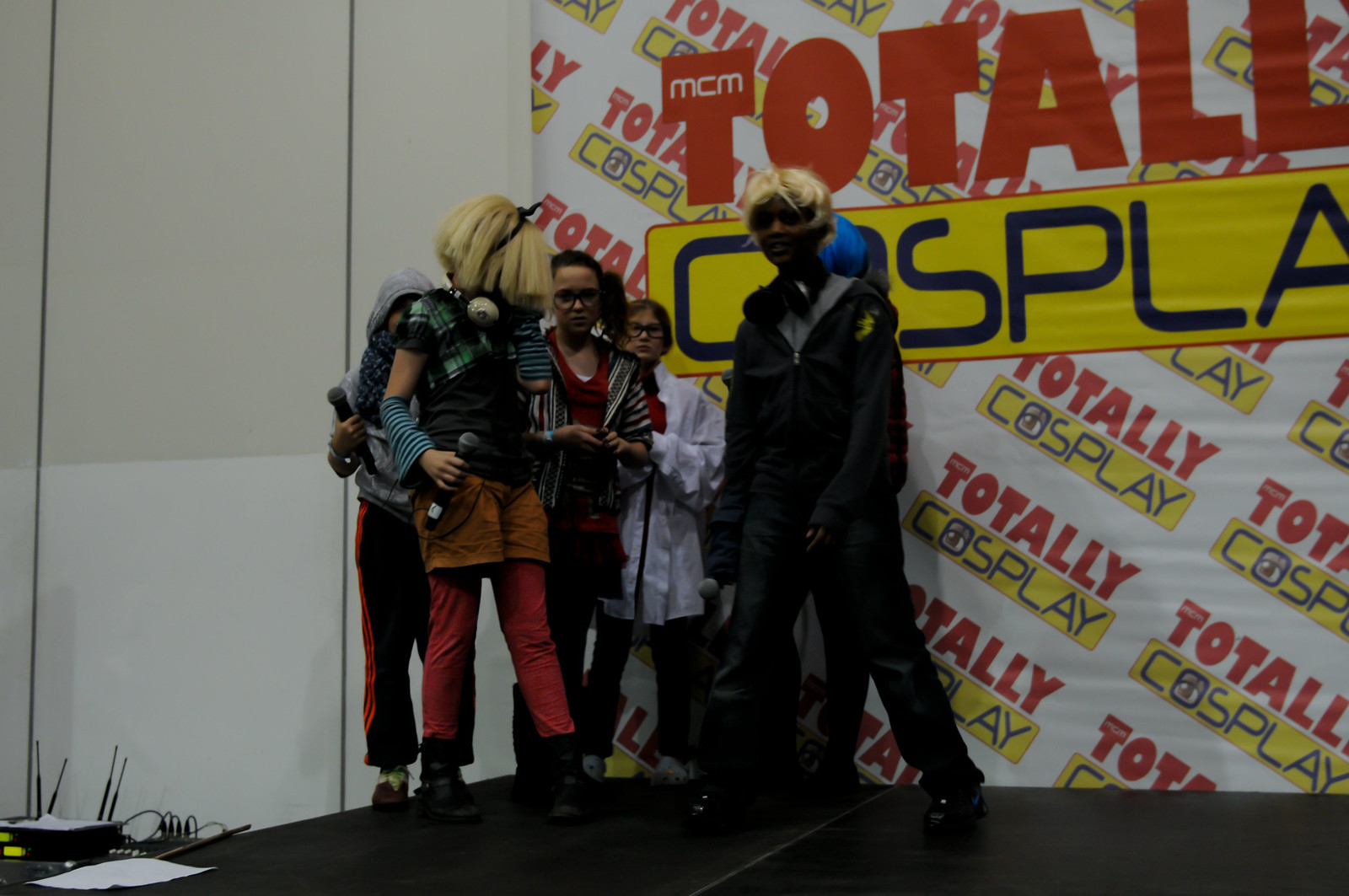The photograph captures a lively scene at a gaming convention titled "Totally Cosplay," prominently displayed in large text across the top right corner of the stage. The word "Totally" is styled in red with the letters "MCM" in white inside the "T," while "Cosplay" is presented in blue within a red rectangle. Below this title, a repeating pattern of the phrase "Totally Cosplay" is visible, adding to a vibrant backdrop. 

On the black stage, a diverse group of six young children, approximately seven to eight years old, stand in various elaborate costumes emulating their favorite gaming characters. At the forefront, a young girl with a blonde wig, dressed in a black shirt, orange shorts, red tights, and tennis shoes, holds a microphone in her right hand. Beside her, a boy wears a black jacket, a blonde wig, and sunglasses. Another child is dressed in a white lab coat over a red shirt, portraying a doctor. 

Towards the back, a child in a lime green hoodie with dark pants stands near another in casual clothing, including a hoodie and headphones, embodying a gamer look. Additionally, a child with blue hair is seen peeking from behind, contributing to the colorful ensemble. The stage is flanked by a mixture of casual attire and more intricate costumes, with electronics visible at the bottom left corner. The white and gray walls of the staging area contrast with the dynamic costumes, underscoring the festive atmosphere of the gaming convention.